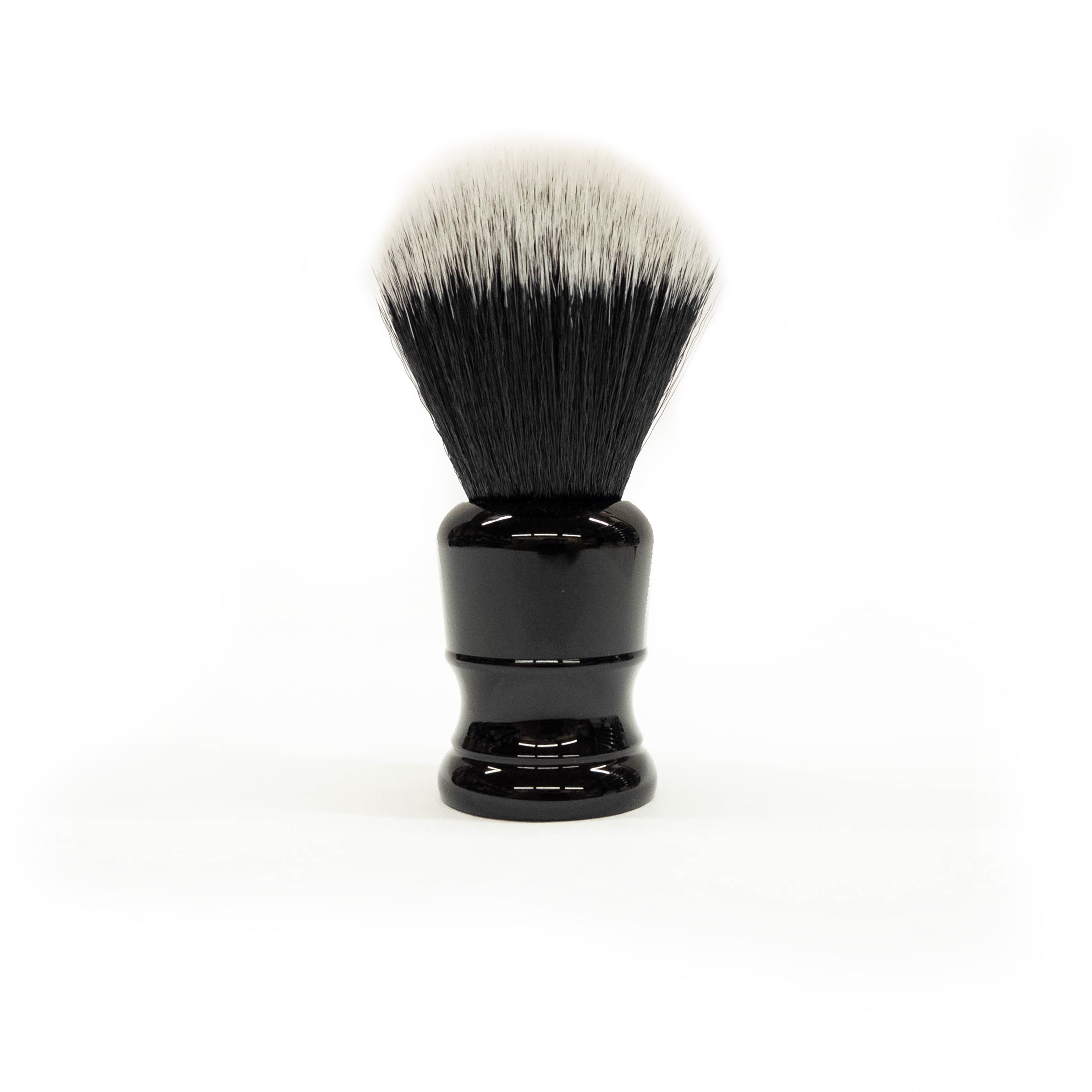The image depicts a makeup brush with a sleek, black, and shiny base that appears to be made of plastic or metal. The brush has a tapered neck that widens at the bottom, resembling the size of a thumb. The entire brush, including the handle and bristles, is about three inches tall, with the base alone being roughly an inch and a half high and an inch across. Its bristles are densely packed and predominantly black, transitioning to white at the tips. The white coloration at the tips suggests recent use, possibly for applying foundation or another makeup product. The background of the image is plain white, providing no additional context or elements, focusing solely on the small, stubby brush reminiscent of those used both in makeup application and barber shops for lathering.